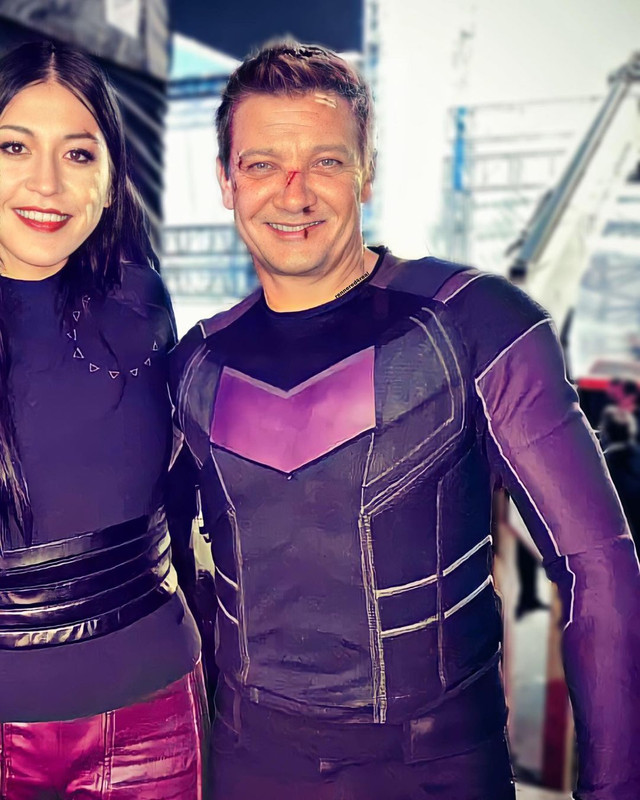This photograph features Jeremy Renner, best known for his role as Hawkeye in the Avengers series, accompanied by an unidentified woman. Both individuals are dressed in eye-catching costumes. Jeremy Renner is depicted in a form-fitting purple suit, characteristic of a superhero or a sci-fi character, prominently occupying most of the frame. The costume includes tight sleeves and a distinctive V-shaped texture on his chest. Notably, Renner has several makeup injuries: a cut on his forehead covered with two small pieces of tape, a horizontal cut at the bridge of his nose with blood trickling, a bit of blood on his lip, and another cut on his right eyebrow also covered with tape.

Standing to Jeremy's left is a woman with long black hair that cascades down to her mid-waist. She sports a tight purple shirt featuring five thin bands around the waist and a circular pattern composed of small triangles on the top left shoulder, resembling a sun. Her outfit is completed with striking hot pink pants that are cut off at the top of the thighs. The woman appears to have a Hispanic background, highlighted by her red lipstick and confident demeanor. Despite the right side of her body being partially out of the frame, her presence adds a complementary dynamic to the image, enhancing the visual narrative of the scene.